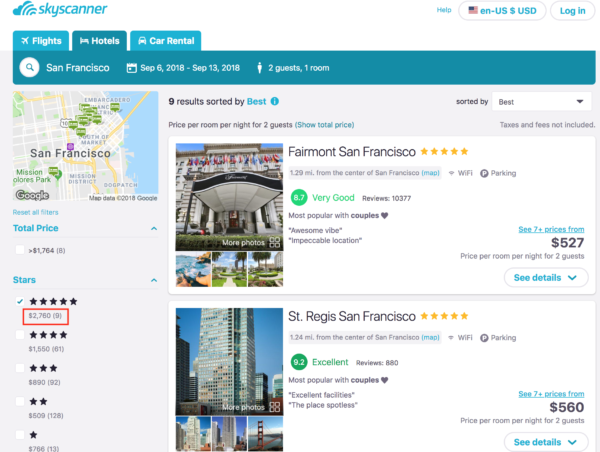The image displays a screenshot of the Skyscanner website, with the Skyscanner logo and name prominently located in the top left corner. To the right, there are options for help, configuring the country and currency, and a login button. Below this header, a blue banner contains several tabs: Hotels, Flights, and Car Rental. The Hotels tab is currently active, focusing on accommodations in San Francisco. Beneath the blue panel, on the left side, there's a map of San Francisco.

The current search appears to be filtered for five-star hotels, displaying nine results. However, only two are visible in the cropped image. The first visible hotel is the Fairmont, San Francisco, which is rated as 'Very Good' based on 10,377 reviews. It is priced at $527 per night for two guests. The second visible hotel is the St. Regis, San Francisco, noted for its 'Excellent' rating, with a typical nightly rate of $560 for two guests.